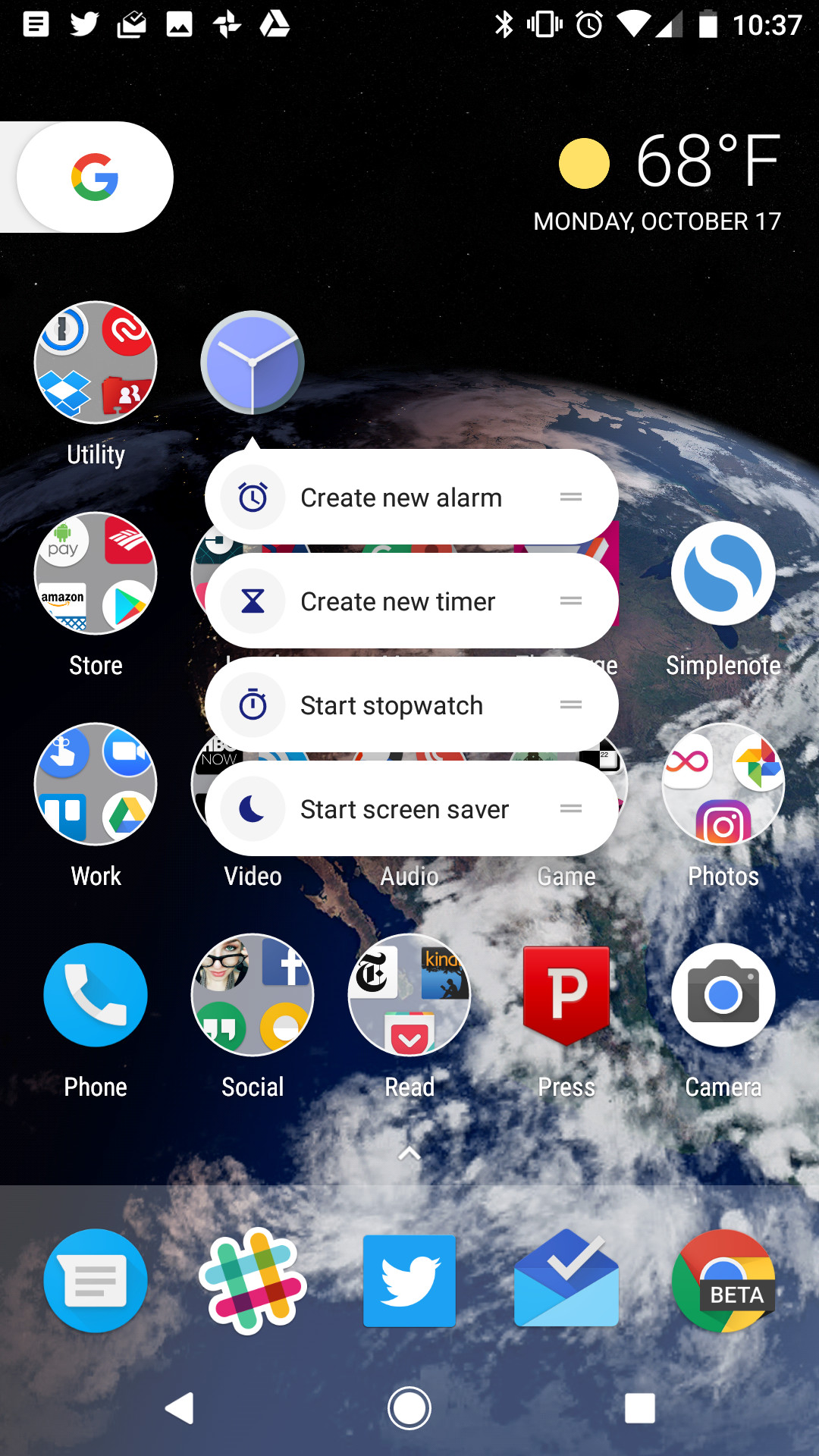This screenshot captures a detailed view of a smartphone's home screen. The status bar at the top displays various icons indicating active features: a text message icon, a Twitter bird icon, an email icon, a photo or screenshot icon, a OneDrive icon, and a Google Photos icon. The Bluetooth is turned on, the phone is set to vibrate, there's an alarm set, and it’s connected to Wi-Fi with a moderate signal strength. The battery is nearly full. The time displayed is 10:37. Just below the time on the top right corner, the current weather is shown with a sun icon, indicating 68 degrees Fahrenheit. The date is displayed as Monday, October 17th. 

In the top left corner, there is a Google search bar, showing only the Google icon. Below this search bar are various app icons and folders. The first row includes a utility folder with additional options visible due to a long press on the alarm icon, which offers options like 'Create new alarm,' 'Create new timer,' 'Start stopwatch,' and 'Start screensaver.' The second row begins with a store icon, followed by three obscured icons, and ends with the SimpleNote app. The third row contains folders labeled as 'Work,' 'Video,' 'Audio,' 'Game,' and 'Photos.' The bottom row displays icons for 'Phone,' 'Social,' 'Read,' 'Press,' and 'Camera.'